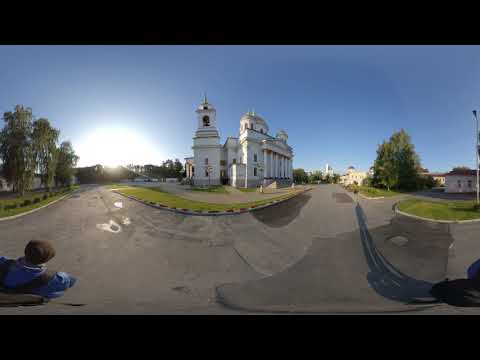This detailed scene combines elements from three descriptions to provide a cohesive and vivid narrative of a complex image. The image primarily represents an outdoor landscape in a town, featuring a prominent and large white building that could be a church, estate, or government building, distinguished by its bell tower and long white columns—a testament to its significance. The building, faced with white marble, stands prominently in the center, with steps leading to what might be an entrance supported by columns.

The photograph is taken from an angle that captures both roads flanking the building. One road curves in from the left, lined with trees and residential-looking structures peeking from behind the foliage. The other road converges from the right, bordered similarly by trees and extending towards some more modern buildings in the distance, suggesting this is a corner of a larger urban area.

The clear sky with bright sunlight coming from the left suggests it is mid to late afternoon. A person with a blue jacket and backpack is visible to the left, adding a human element to the otherwise architectural and natural scene. The image’s edges, particularly the lower left corner, are slightly distorted, hinting at a wide-angle photograph compressed to fit the frame.

In the lower left-hand corner of the scene lies a curious, unidentifiable object, possibly a teddy bear with a material that appears blue. It stands out against the otherwise detailed and realistic background, making it an interesting focal point of mystery amidst the structured environment.

The overall composition with the roads, trees, modern and classic architectural elements, combined with clear, bright skies, renders a rich and detailed photographic narrative without text, emphasizing the centrality and prominence of the white building.